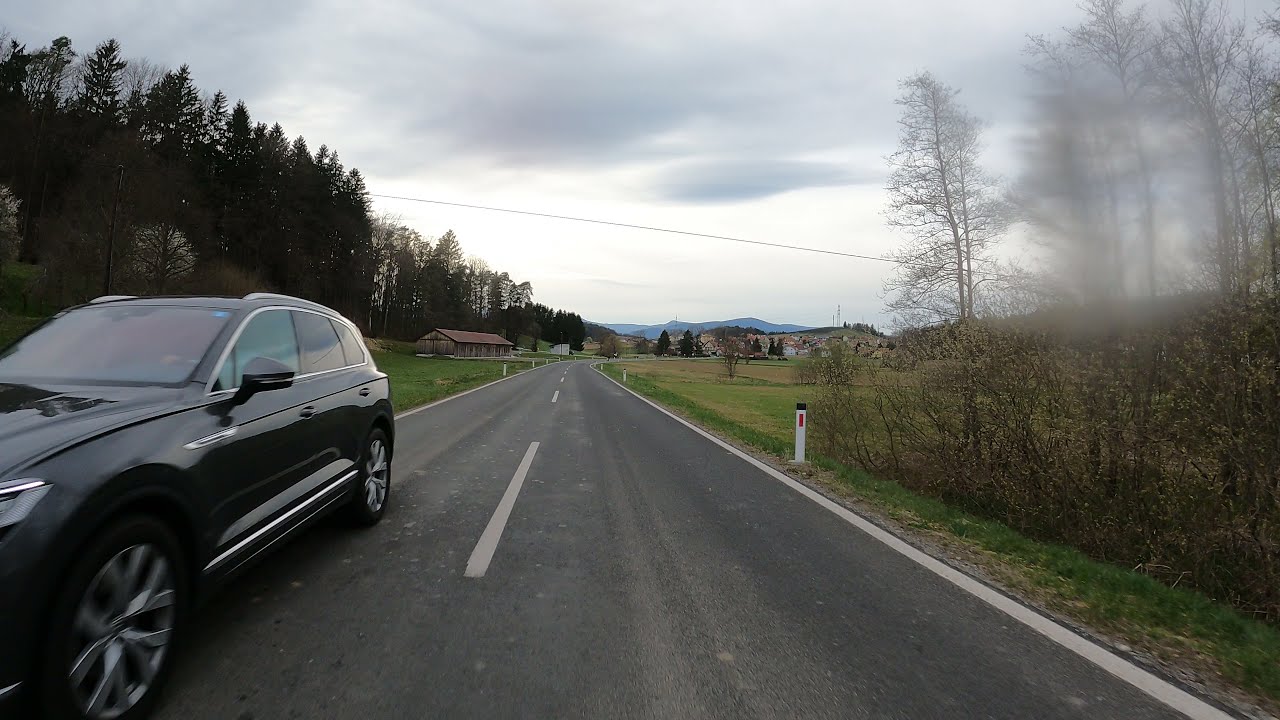The image captures an outdoor scene along a two-lane road during the daytime. A black SUV is driving towards the viewer, positioned in the opposite lane from the person taking the photograph. The road, which initially runs straight and curves towards the right, features white dotted lines down the middle and solid white lines marking its edges. Both sides of the road are bordered by grassy areas, with a noticeable slope and some farmland visible on the right. White poles with red reflectors line the road for better visibility. 

The backdrop includes a mix of tall pine trees and some leafless deciduous trees, with a blurred section of trees suggesting motion. In the far distance, a small town with conical or triangular-roofed houses is visible, framed by a range of mountains. Overhead, the sky is mostly cloudy with a mix of dark and lighter clouds, adding a somewhat gloomy atmosphere to the scene. Additionally, power lines span the sky, contributing to the overall detail of this rural landscape.